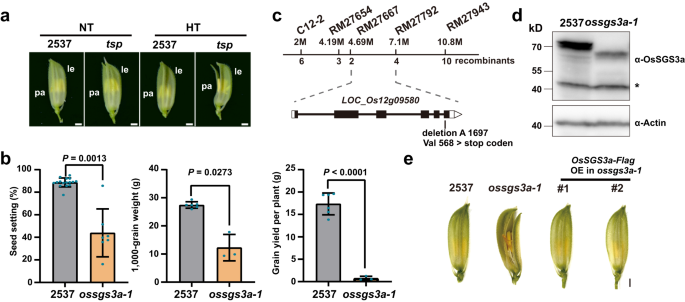The image is a detailed scientific diagram, possibly related to agriculture or horticulture, presented in a landscape format divided into five sections labeled A, B, C, D, and E. Each section offers distinct information, contributing to the overall understanding of the graphic.

Section A, in the upper left, depicts plant stems at various stages of opening, with subtle details under a black background. Section B features three bar graphs labeled with “2537” in grey and "OSSGS3A-1" in salmon pink, providing comparative data points. Section C includes line graphs with specific numerical markers—C12, RM27654, and RM27667—emphasizing detailed data trends. Section D is described as less clear, with blurry images that are difficult to decipher. Section E mirrors Section A, showcasing plants in different stages of both opening and closing.

Notably, sections of the image include noteworthy formulas such as NT/2537 TSP and HT/2537 TSP. Additionally, there are four pictures resembling green leaves or plant parts against a black background, marked with "P-A-L-E" in white text. The bottom left of the image reveals more bar graphs with extensive information, while the bottom right contains a cluster of four leaves, central to the diagram's visual narrative.